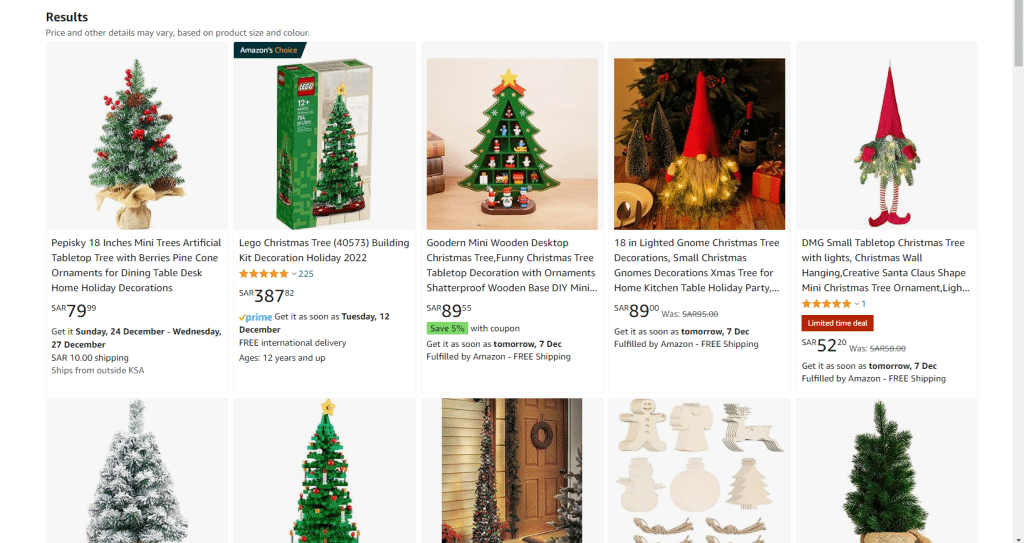The image appears to be a screenshot from an Amazon webpage showcasing a variety of decorative Christmas trees. Starting from the top left, the first item is an 18-inch artificial tabletop Christmas tree priced at SAR 79.99. Next to it on the right, marked as Amazon's Choice, is a Lego Christmas tree available for SAR 387.82 with Prime shipping. Following this, to the right, is a Goodberg mini wooden desktop Christmas tree priced at SAR 89.55.

Continuing to the right, there is an item that does not resemble a Christmas tree but instead features a red hat and is priced at SAR 89. Directly to its right is a similar item, also adorned with a red hat but additionally featuring legs and red shoes, priced at SAR 52.20.

Beneath these primary products, five other items are partially visible: a white Christmas tree, a green Christmas tree, an outdoor tree, a set of cookie cutters, and another tree with a remarkably realistic appearance.